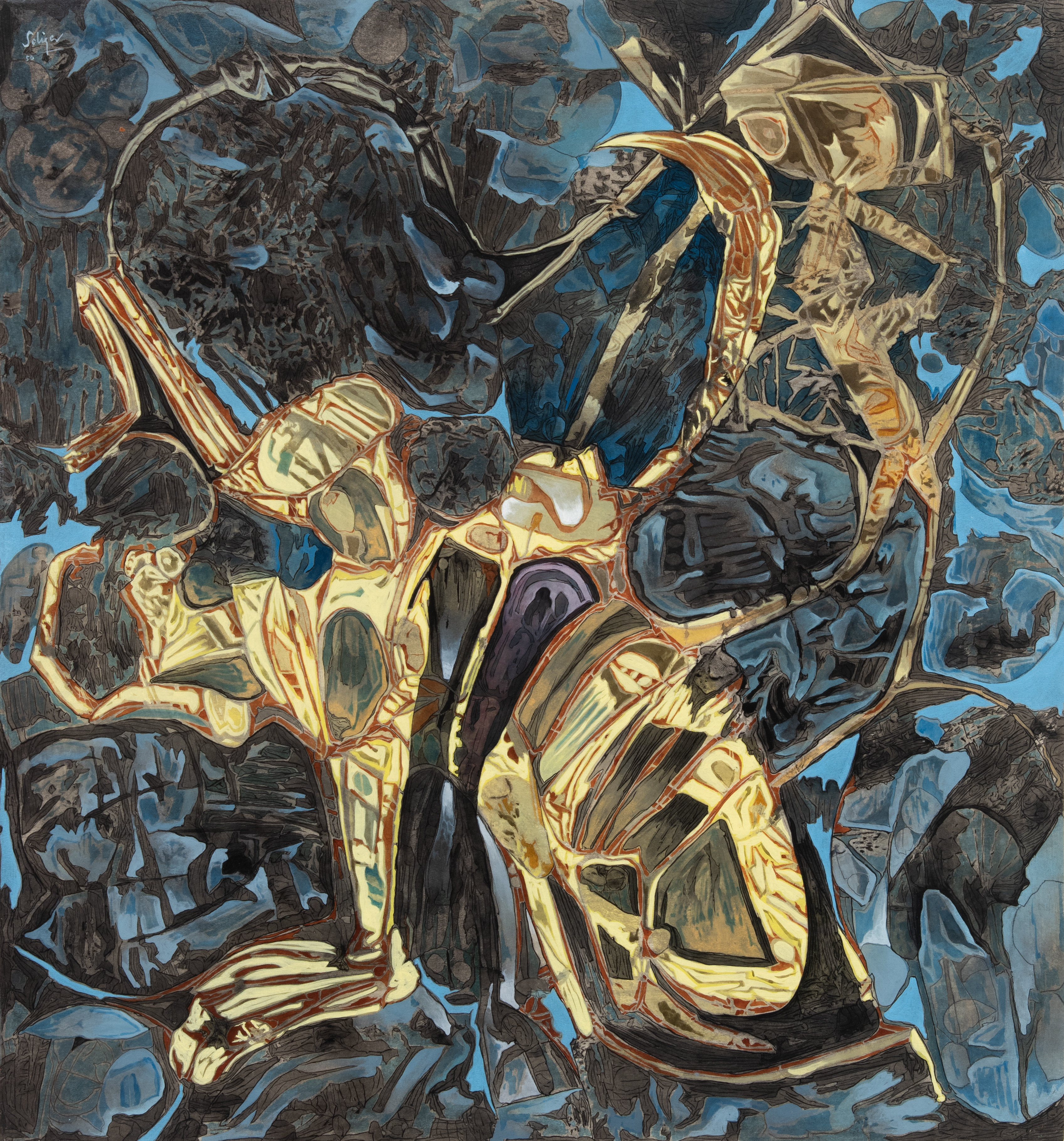The image showcases an abstract painting dominated by various shades of blue, metallic blue, gold, gray, and black. At the center, there is a complex, almost mechanical-looking figure, primarily yellowish-gold, resembling a cross between a dog and a scorpion with its distinct features like a paw, perked ears, a possible beak, and multiple limb-like projections. This primary figure appears to be facing a smaller, more scorpion-like entity on the far right. The backdrop is an intricate combination of light blue with darker blobs of graphite purple-gray, adding depth and contrast to the surreal composition. Overall, the artwork exudes a unique, original style with interconnected, peculiar shapes and a blend of abstract elements, making it quite evocative and open to interpretation.